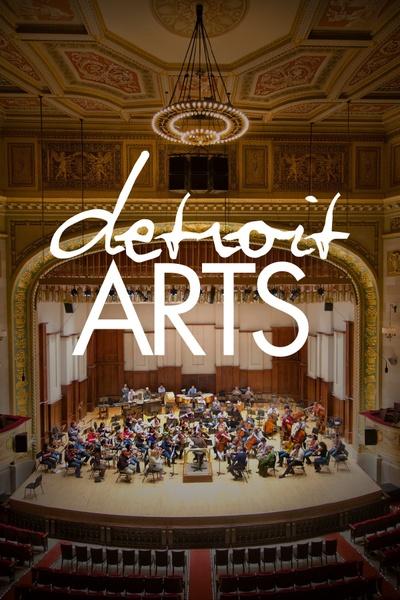This image showcases a historic theater with "Detroit Arts" prominently displayed in the center. The theater boasts an ornate ceiling with gold trim and angelic artwork, alongside a grand chandelier. A wooden stage, positioned centrally, is adorned with numerous musicians seated and playing various instruments. The seating area for the audience is well-organized with rows of chairs separated by red carpeted pathways. The stage is set against a backdrop of brown and white walls, and rich drapes and curtains enrich the visual appeal. The intricate architecture and the mix of warm colors like tan, brown, red, and beige add to the elegance of the scene. The photo, potentially digitally enhanced or artistically rendered, captures the detailed and vibrant atmosphere of an indoor musical performance, viewed from an elevated perspective.